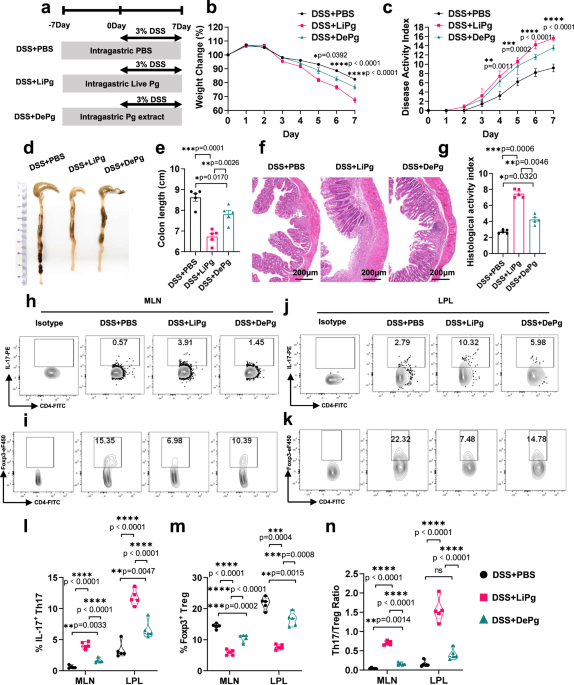The image depicts a comprehensive scientific study featuring a series of graphs, charts, and figures labeled alphabetically from A to N. Key terms like DSS, PBS, DEPG, and LIPG are prevalent throughout, illustrating different experimental conditions and outcomes. At the top right, there are two line graphs, while three bar graphs occupy the bottom section. Above the bottom graphs, 16 small x-ray figures are displayed. The middle section includes various scales on figures of microscopic entities, highlighted by a distinctly colored purple and yellow image. The study appears to focus on the histological activity index and disease metrics like weight change, disease activity index, and mass sizes, with numerous data points indicating changes over time. The black-and-white color scheme punctuates the more detailed elements, providing a visually detailed and data-rich image of scientific research outcomes.